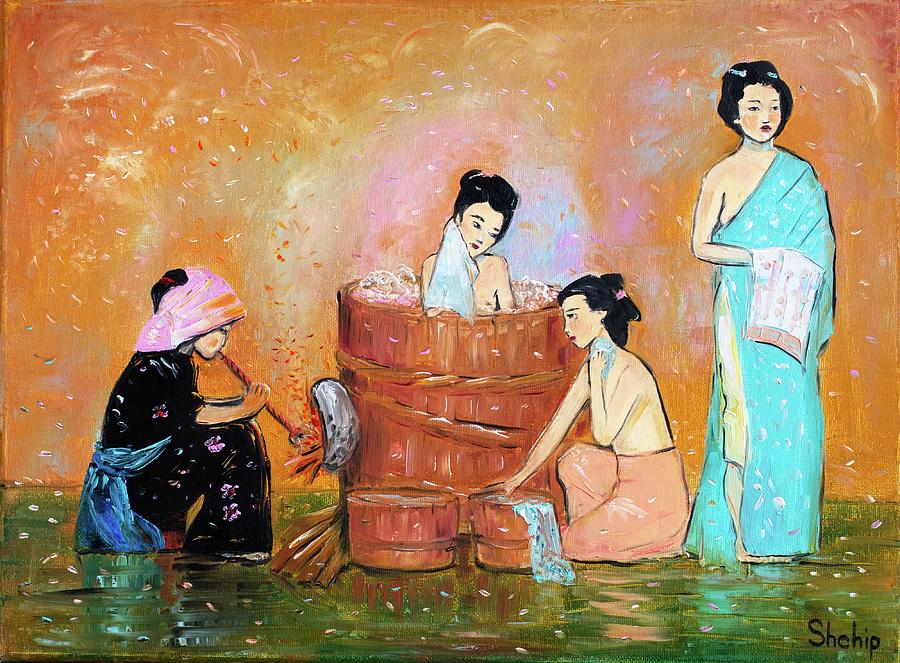This painting, likely of Chinese origin, portrays a detailed and intimate scene of a woman bathing in a wooden tub at its center. The woman in the tub, with her black hair tied up, gently presses a wash towel to her right cheek amidst bubbles in the water. Before the tub lies a wooden stave barrel, accompanied by two smaller buckets. To the right, a kneeling woman tends to her tasks, while behind her, a standing woman in a blue wrap adorned with white dots holds a towel in her right hand. This standing woman, also with tied-up black hair, displays a slightly indifferent expression. On the left side of the scene, a woman in black floral-patterned attire with a blue sash and a pink hair covering, sits on a box, seemingly playing a pipe. The setting is enriched by a green, reflective floor and a peach-colored wall with intricate dot and curve patterns, adding to the painting’s vivid yet serene ambiance. The painting’s base features an inscription, "SheHIP," rendered in black.